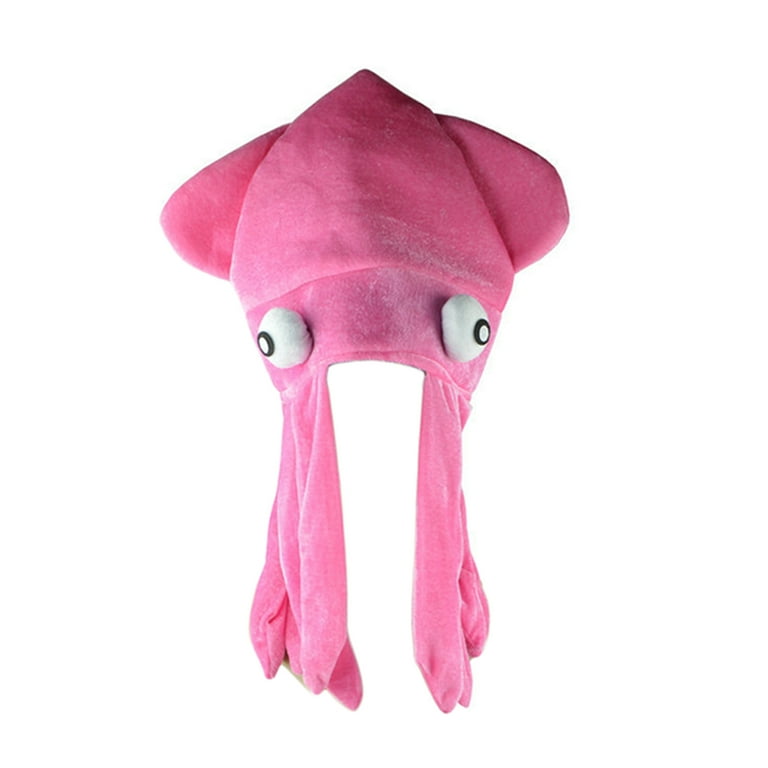This image is a color photograph of a whimsical, pink octopus hat, designed like a kid's winter hat or "boggin." The hat is crafted from a soft, fleece-like fabric and features a playful and cartoon-like appearance. It has a peaked top and is adorned with large, rounded ears that extend down the sides.

At the center of the hat, just below the peak, are two prominent, googly eyes. These eyes are large and white, each with a black circle and two smaller white dots within the black circles, creating a lively and animated expression. The eyes are connected by a pink strip of fabric.

The hat also includes octopus tentacles, which dangle down from beneath the eyes. There are four tentacles on the left side and two on the right, all made from the same pink fabric as the rest of the hat. The overall design is reminiscent of the iconic hat worn by Louise Belcher from the cartoon "Bob's Burgers," but with added googly eyes for extra charm. The background of the image is plain white, with no additional elements or borders, allowing the quirky, detailed design of the octopus hat to stand out.